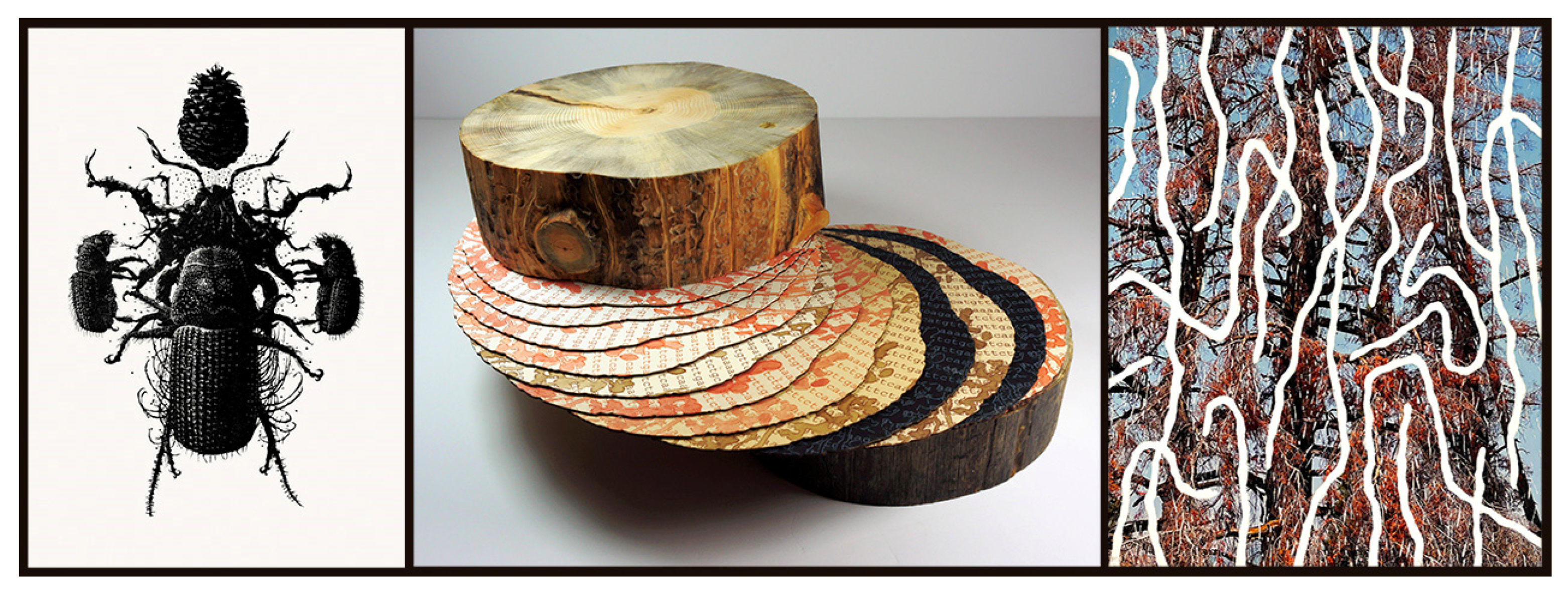This is a three-section horizontal photo collage with varying image sizes. On the left, against a white background, there's a detailed black beetle illustration showcasing front, top, and side views. Two smaller beetles flanking the central beetle suggest dynamic interaction, while the black and white palette emphasizes the intricate forms. The middle section features a cross-section slab of a tree trunk on a gray background, with fine, almost paper-thin layers between top and bottom trunks. These layers display orange and white colorings resembling tree rings, enriched with gold, red, and brown tones. The right section portrays a possibly dying evergreen tree with red leaves and a blue sky backdrop. Overlaying this image is a pattern of white squiggly lines, mimicking boring lines, which adds a textured, bark-like effect running from top to bottom.